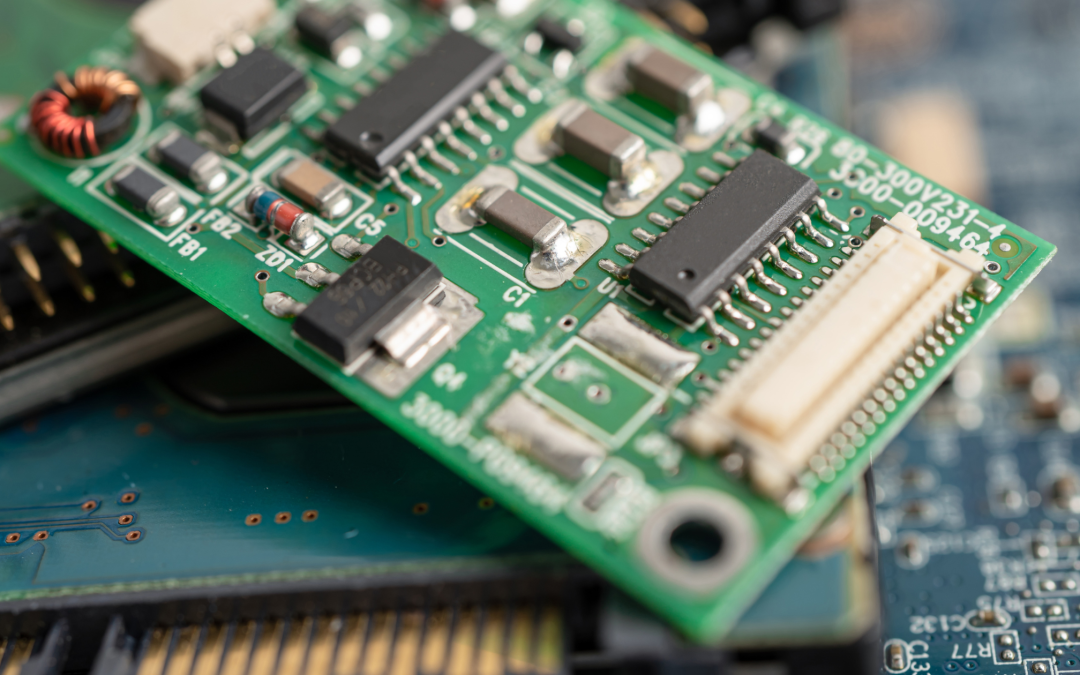This is a detailed close-up photograph of a green motherboard, prominently featuring intricate circuitry. The motherboard is arranged from the upper left to the bottom right of the image, and it sits atop a stack of other computer components, which are blue, gold, and dark in color. The board is populated with various silver and black components, including multiple chips in brown, black, and light tan. A notable feature in the top left corner is a black circle with a copper coil, while the bottom right features a white circle with a black center. Scattered across the board are printed numbers and letters such as "300V231-4" and "3000-009464." The image, captured in landscape mode, focuses so closely on the components that it obscures the broader environment, giving an impression of interior lighting.